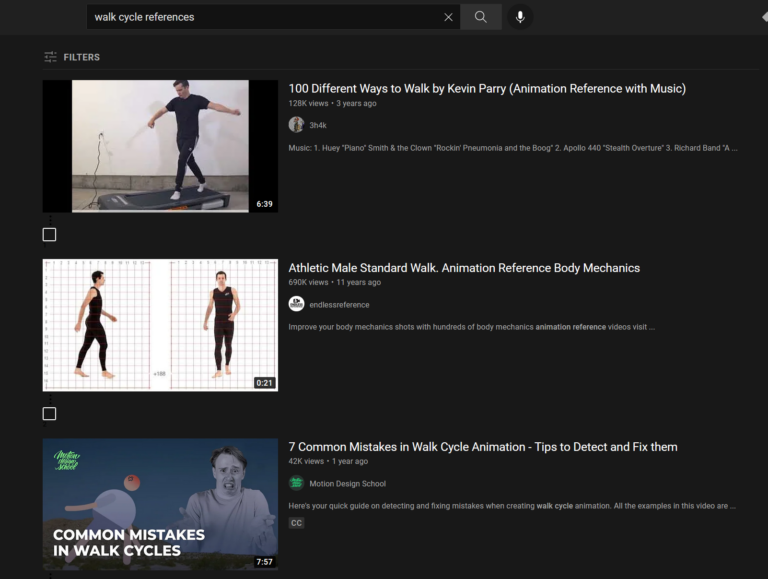The image depicts a black-background webpage focused on different exercise videos specifically for walk cycle references. At the top, there’s a filter section for sorting the content. On the left side, there are three vertically aligned videos, each showing their duration and a preview image, while on the right side, there are detailed descriptions providing more information about each video.

1. The first video features a man walking on a treadmill that lacks balancing bars, indicative of a more natural walking motion. The video is titled "100 Different Ways to Walk" by Kevin Perry and has a duration of 6 minutes and 39 seconds. It is categorized as an animation reference with accompanying music. This video has garnered 128K views and was uploaded three years ago. The profile picture is visible, and the music tracks listed are "Rockin' Pneumonia and the Boogie Woogie Flu" by Huey "Piano" Smith and "Stealth Overture" by Apollo 440 with Richard Band.

2. The second video is titled "Athletic Male Standard Walk Animation Reference: Body Mechanics." It focuses on demonstrating the standard walking mechanics of an athletic male, intended as an animation reference for artists and animators.

3. The third video is titled "Seven Common Mistakes in Walk Cycle Animations: Tips to Detect and Fix Them." This tutorial aims to educate on the frequent errors in animating walk cycles and offers solutions to improve the accuracy and fluidity of these animations.

This detailed layout provides animators and artists with a variety of visual and instructional resources to perfect their walk cycle animations.